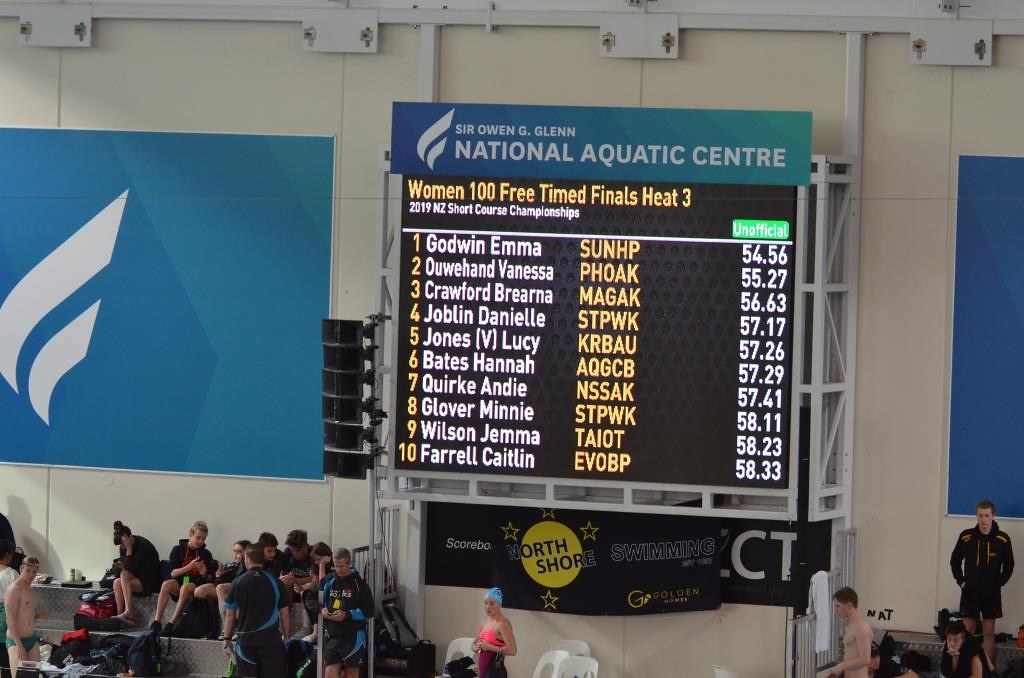This detailed photograph captures a moment at the 2019 NZ Short Course Championships held at the Sir Owen G. Glenn National Aquatic Center. In the foreground, a swimmer stands in a swimsuit and swim cap, indicative of a women's swimming competition. The focal point of the image is an illuminated scoreboard displaying the results of the Women’s 100 Free Timed Finals Heat 3. Topping the list is Emma Goodwin with a time of 54.56, while the 10th position is held by Kaitlin Farrell at 58.33. The scoreboard, which has white text against a blue background, is flanked by blue posters and bears the title of the event and venue. The scene is set in a bustling aquatic center, with men and women, some in swim attire and others in gym jackets, seated on the bleachers below the scoreboard. Their presence adds to the lively atmosphere of this competitive swim meet.